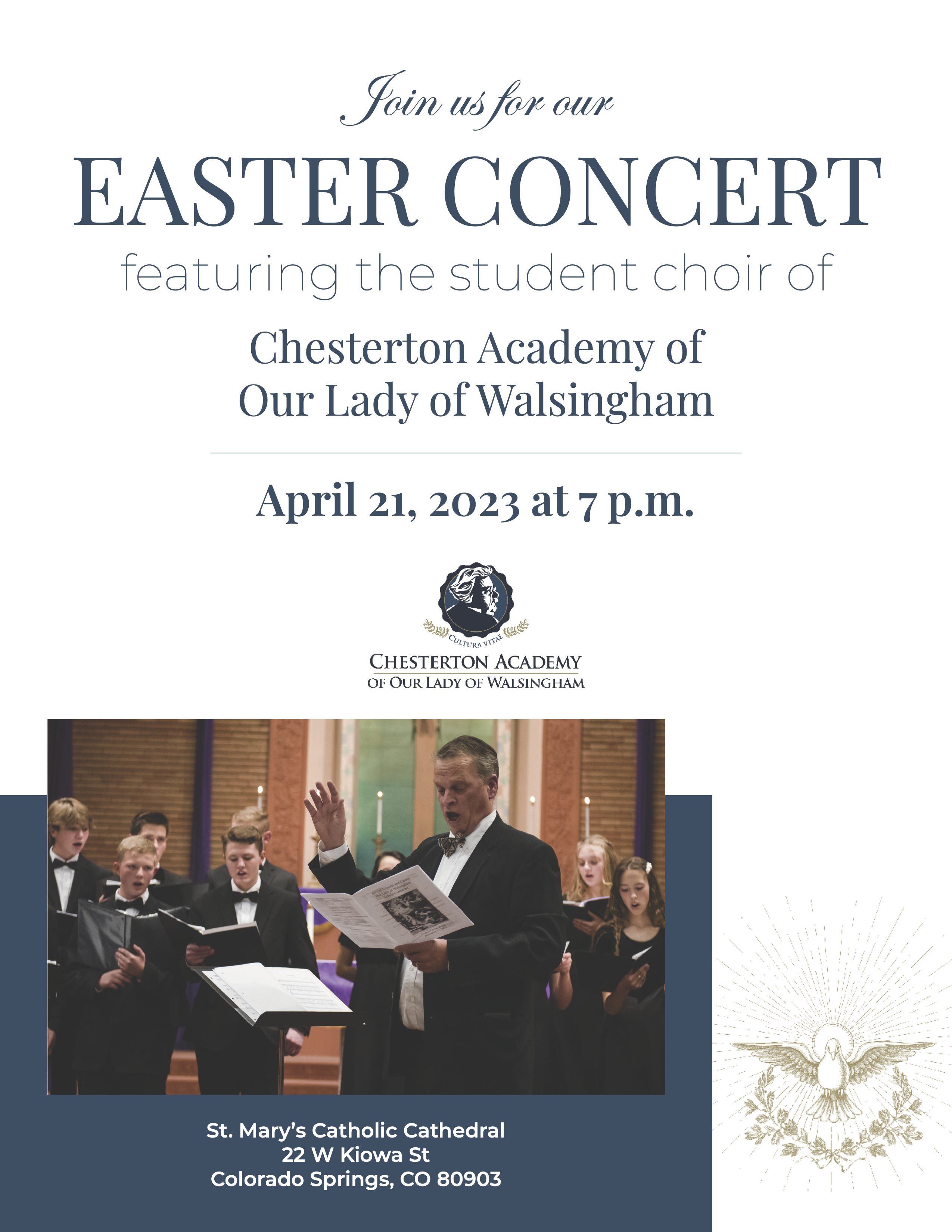The advertisement flyer for the Easter concert at St. Mary's Catholic Cathedral is predominantly white, adorned with a mix of fonts and vibrant colors. At the top, in a dark grayish-blue cursive font, it reads, "Join us for our," followed by a large serif font highlighting "Easter concert." Beneath this, thin, small sans serif text introduces the event, "featuring the Student Choir of Chesterton Academy of Our Lady of Walsingham," with additional details such as the date and time, "April 21, 2023, at 7 p.m."

The image at the bottom of the flyer showcases the choir in performance. The foreground features an older man with a bald head and a tenor voice, dressed in formal attire, including white shirts, bow ties, shoes, and smart trousers. Behind him are younger teens holding books, intently singing, forming the main body of the choir. The background reveals the majestic altar of St. Mary's Catholic Cathedral, adorned with candles and gothic detailing. Enclosed within a dark blue-gray box, the text at the bottom provides the venue's specifics: "St. Mary's Catholic Cathedral, 22 W Kiowa Street, Colorado Springs, CO, 80903." The flyer conveys a sense of elegance and reverence, reflecting the significance of the Easter concert event.